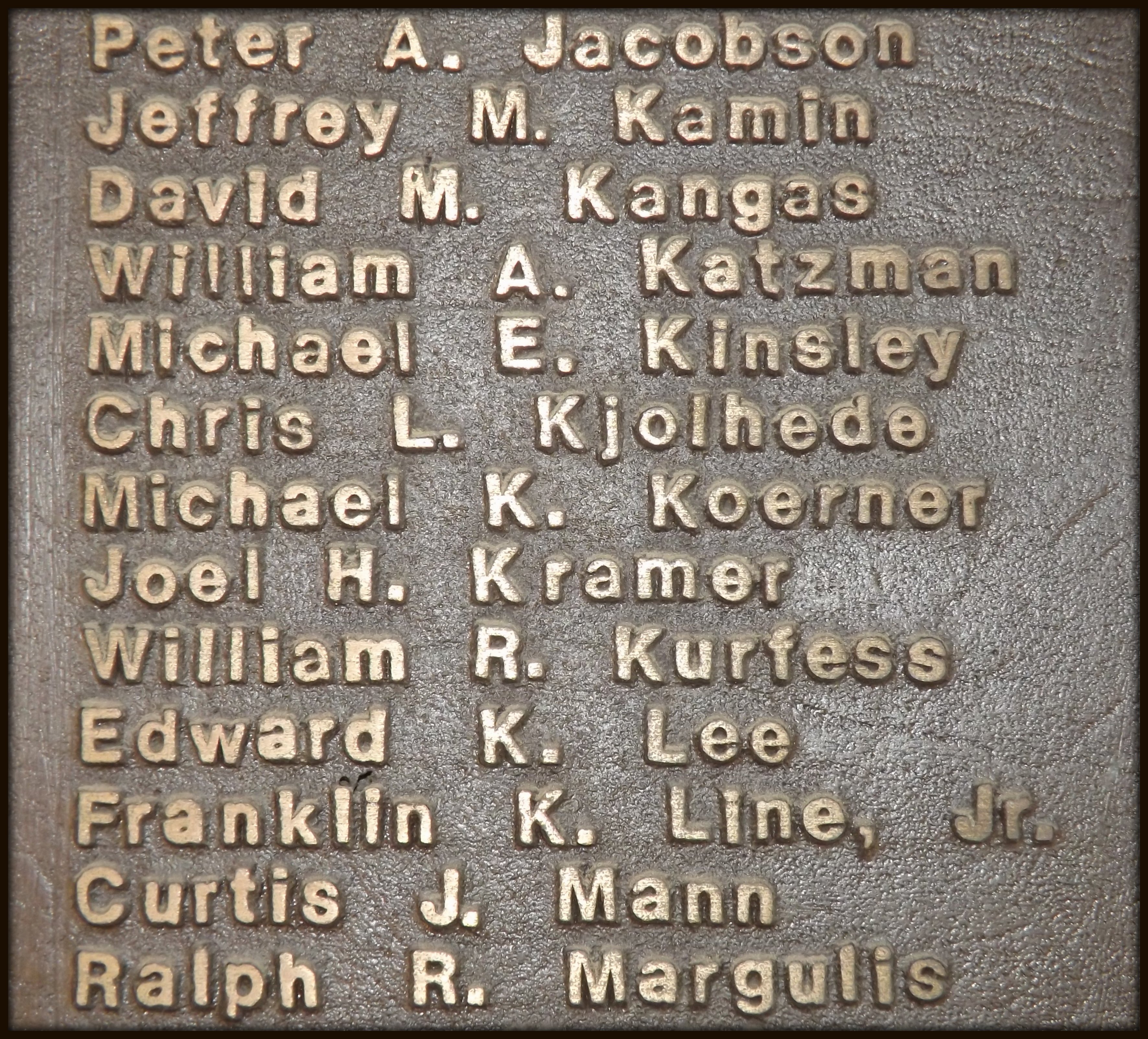The image showcases a weathered bronze plaque with names etched in bronze letters, appearing to be a memorial plaque from the Cranbrook School. This plaque, titled "Alumni Court," lists the names of members of the class of 1968, including Edward K. Lee, Franklin K. Lyne Jr., Curtis J. Mann, and Ralph R. Margulis. The plaque shows signs of age with visible grooves and scratches, indicating its historical significance. From top to bottom, the detailed list of names includes Peter A. Jacobson, Jeffrey M. Kameen, David M. Kongis, William A. Katzman, Michael E. Kinsley, Chris L. Kjolhed, Michael K. Korner, Joel H. Kramer, William R. Kerfes, Edward K. Lee, Franklin K. Lyne Jr., Curtis J. Mann, and Ralph R. Margulis.